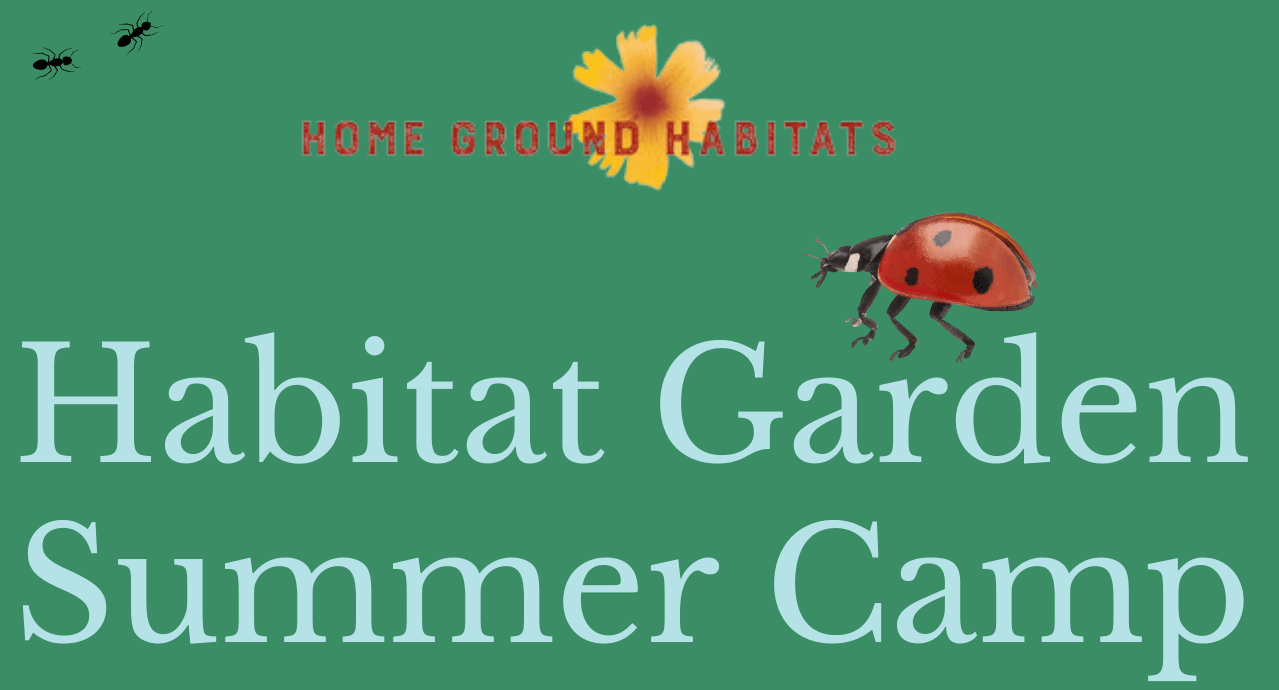The image resembles a book cover or an advertisement for a summer camp program. The background is a detailed green with a light, sage green hue. Prominently featured at the top center is a yellow flower with vibrant yellow petals and a bright red center. In the upper left-hand corner, two small black ants can be seen, adding a lively touch to the design. Towards the middle right of the image, there's a real photograph of a ladybug with a shiny red shell adorned with black spots, skinny black legs, and a distinct white strip on the underside of its head. The text is prominently displayed, with "Homeground Habitats" in red letters at the top against the yellow flower, and "Habitat Garden Summer Camp" in light blue letters at the bottom, making the purpose of the image clear and inviting.